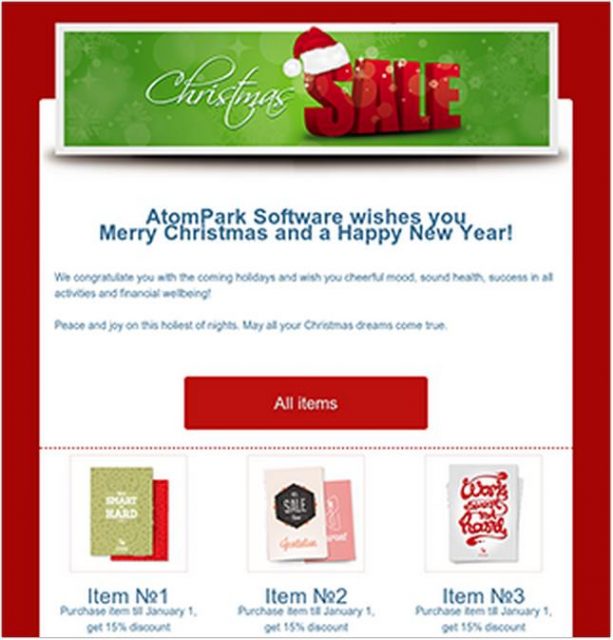**Detailed Caption:**

The screenshot showcases a festive Christmas sale promotion from an e-commerce website. The background is predominantly red, creating a vibrant and holiday-themed aesthetic. At the top of the image, there is a green banner adorned with transparent snowflakes, giving it a wintry feel. The word "Christmas" is written in white letters on the banner, while the word "SALE" stands out in bold red letters. To add a touch of whimsy, a Santa hat playfully sits atop the "S" in "SALE." The green banner has a white outline and a subtle shadow beneath it, adding depth and dimension to the design. 

Below the banner, there is a white box with a festive greeting from "Adam Park Software," wishing viewers a Merry Christmas and a Happy New Year. This message is accompanied by some text in blue, likely elaborating on the sale or providing additional information. At the bottom of this white box is a prominent red button labeled "All Items," inviting users to view the full selection. This button is underscored by a dashed line, adding a visual break.

The lower part of the screenshot displays three featured items that resemble greeting cards. The first card, labeled "Item Number One," appears to have a glittery cover, making it sparkle elegantly. "Item Number Two" is characterized by a pink cover, overlaid with a sale image, likely indicating a special discount. The third item stands out with its white background and red text, providing a clear and festive design. Together, these elements combine to create a visually appealing and festive promotional image, perfect for enticing shoppers during the holiday season.